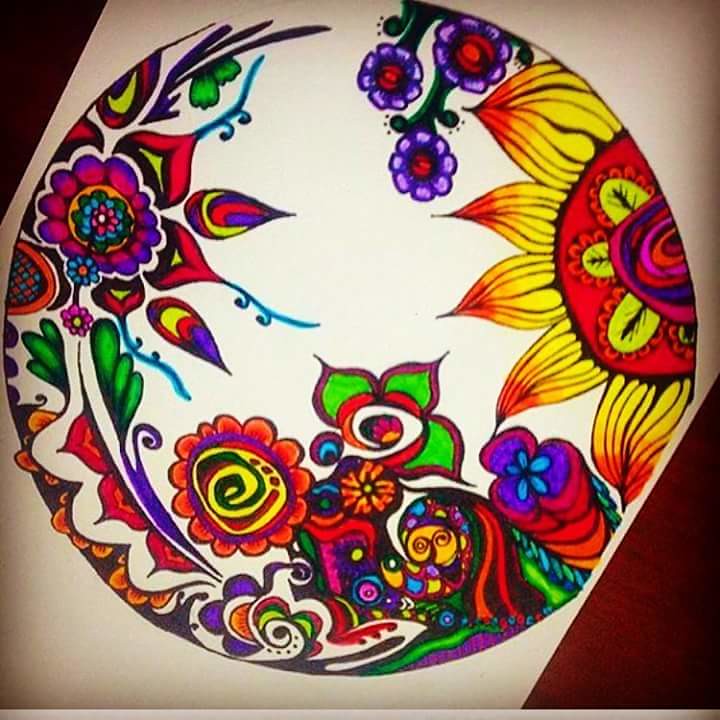The image is a digital illustration that mimics a colorful tattoo, potentially sketched for placement on someone's arm or leg. The main feature is an imperfect circular design set against a skin-tone background, suggesting a tattoo concept. The circle spans about 80% of the frame and has a slightly flattened right side with a small section missing from the top left, between the 10 o'clock and 12 o'clock positions. Inside the circle, the white base is adorned with an array of vividly colored flowers and patterns.

Starting with the prominent flower on the right side, it is a large, half-visible bloom with a predominantly red center and layered, rainbow-like rings of pink, blue, and orange. The petals of this flower are yellow with red tips and black veins, giving an impression of sun rays emanating outward. Other smaller flowers, in shades of purple, blue, green, and orange, are interspersed throughout the design. Among them are purple flowers with dark green stems and red accents, enhancing the intricate details.

The artwork also features abstract elements open to interpretation, such as yellow petal-like forms on the right that could symbolize sun rays or floral petals. These elements are complemented by delicate, ornate designs that loop and swirl around the composition, emphasizing the hand-painted, intricate nature of the piece.

Overall, the detailed and colorful imagery combined with the skin-toned background creates a compelling representation of a potential tattoo, rich in personal significance and artistic expression.